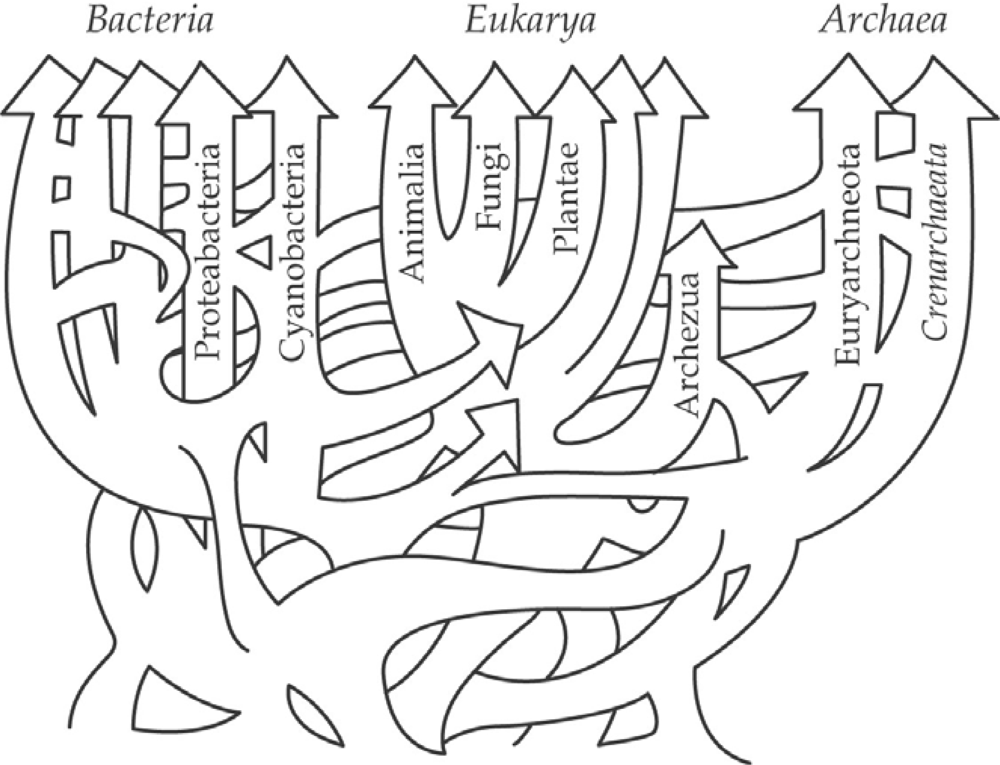The illustration depicts a complex evolutionary diagram set against a solid white background, showcasing the interconnected nature of three main domains of life: Bacteria, Eukarya, and Archaea. Each domain is represented by columns with intricate, intertwining arrows that both connect and diverge, illustrating their relationships and evolutionary pathways.

At the top, the word "Bacteria" is highlighted with multiple arrows underneath, each labelled with terms like "Proteobacteria" and "Cyanobacteria," pointing upwards and towards other columns. The middle column, titled "Eukarya," also has arrows branching upwards to indicate different kingdoms such as "Animalia," "Fungi," and "Plantae." The rightmost column, labeled "Archaea," features arrows leading to "Euryarchaeota" and "Crenarchaeota," demonstrating their subdivisions. 

The arrows not only ascend from each column but also cross-connect, emphasizing the complex and intertwined nature of evolutionary relationships. Each term is clearly marked, contributing to the depth and clarity of the illustration.